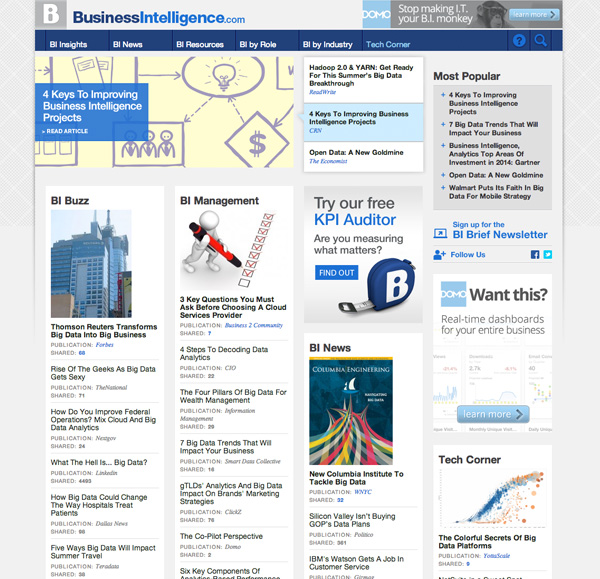Here’s a cleaned-up and detailed caption for the described image:

---

**Descriptive Caption:**

The screenshot is from BusinessIntelligence.com, as indicated by the text in the top left corner. At the top right, a banner reads, "Stop making IT your BI monkey, learn more," and features a photograph of a chimpanzee wearing sunglasses. Below this, the navigation menu includes the tabs: BI Insights, BI News, BI Resources, BI by Role, BI by Industry, Tech Corner, Help, and Search. 

Several headlines and accompanying images are prominently displayed throughout the page. Notable articles include "Four Keys to Improving Business Intelligence Projects," "Hadoop 2.0 and Yarn: Get Ready for This Summer's Big Data Breakthrough," and "Open Data: A New Gold Mine." 

A photograph of a skyscraper accompanies the news piece "Thompson Reuters Transforms Big Data into Big Business." Another key article, "Rise of the Geeks: Big Data Gets Sexy," explores the societal impact of data. Further headlines delve into industry-specific uses of big data, such as "How Big Data Could Change the Way Hospitals Treat Patients" and "Five Ways Big Data Will Impact Summer Travel."

The page also features a drawing of a person holding a pen, checking off a long row of boxes, illustrating the article "BI Management: Three Key Questions You Must Ask Before Choosing a Cloud Services Provider." Other prominent topics include "Four Steps to Decoding Data Analytics," "The Four Pillars of Big Data for Wealth Management," and "Seven Big Data Trends That Will Impact Your Business."

Towards the bottom, a cut-off headline begins with "Six Key Components of..." while a promo recommends users to "Try our Free KPI Auditor," with an image of a blue and white tape measure. Below this, recent "BI News" includes pieces like "New Columbia Institute to Tackle Big Data," "Silicon Valley Isn't Buying GOP's Data Plans," and "IBM's Watson Gets a Job in Customer Service."

Popular articles listed are "Four Keys to Improving Business Intelligence Projects," "Seven Big Data Trends That Will Impact Your Business," and "Walmart Puts Its Faith in Big Data for Mobile Strategy." Additionally, users are invited to sign up for the "BI Brief" newsletter and follow the site on Facebook and Twitter. An attractive offer for "Real-Time Dashboards for Your Entire Business" is displayed alongside the vibrant "Tech Corner" section, titled "The Colorful Secrets of Big Data Platforms."

---

This caption thoroughly describes the content and layout of the screenshot, providing a detailed overview of the key elements presented.